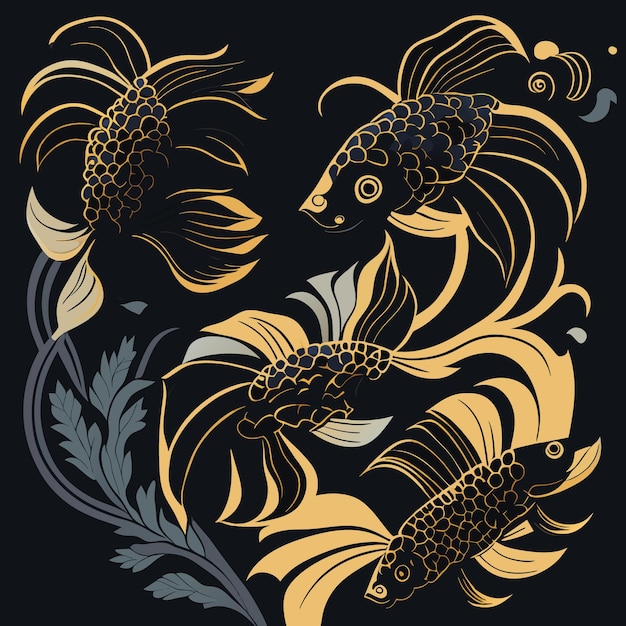This artwork features a dark, almost black background that starkly contrasts with the vivid, light colors used in the foreground elements. The scene appears to be underwater, showcasing aquatic life and flora. Central to the image are several intricately designed fish, rendered in a striking gold, with some possessing long golden tassels or tails. Notably, the fish at the bottom right is unique with two heads. The fish in the center is facing away, emphasizing its long gold tassels, and similar fish can be seen at the top left and top right. The underwater vegetation, located along the left side and bottom, consists of plants with grayish-blue hues and flowers and leaves that are a yellowish gold. The detailed and contrasting elements create a visually captivating underwater tableau.